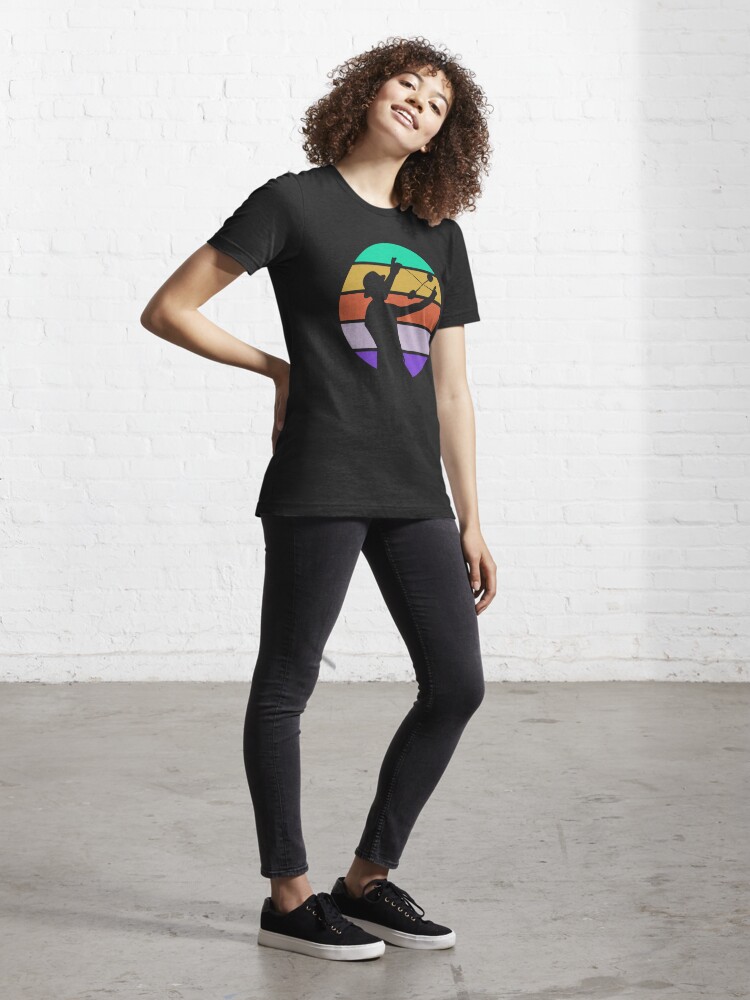This photograph captures a tall, young woman with frizzy brown, shoulder-length hair, casually standing in a room with a white painted brick wall and a bare, concrete floor that reflects her shadow. She has a light to medium Caucasian skin tone and her head is slightly tilted to the left side with a subtle, open-mouthed smile that reveals her teeth. One hand rests on her back right hip, and she is dressed in a black, short-sleeved t-shirt featuring a circular design. The circle showcases a spectrum of colors: green at the top, followed by yellow, orange, lavender, and medium purple at the bottom. At the center of this design is the silhouette of a musician wearing a hat, holding a microphone. She pairs the t-shirt with tight-fitting black pants and black sneakers with black laces and white soles. The overall look reveals a relaxed yet stylish appearance.